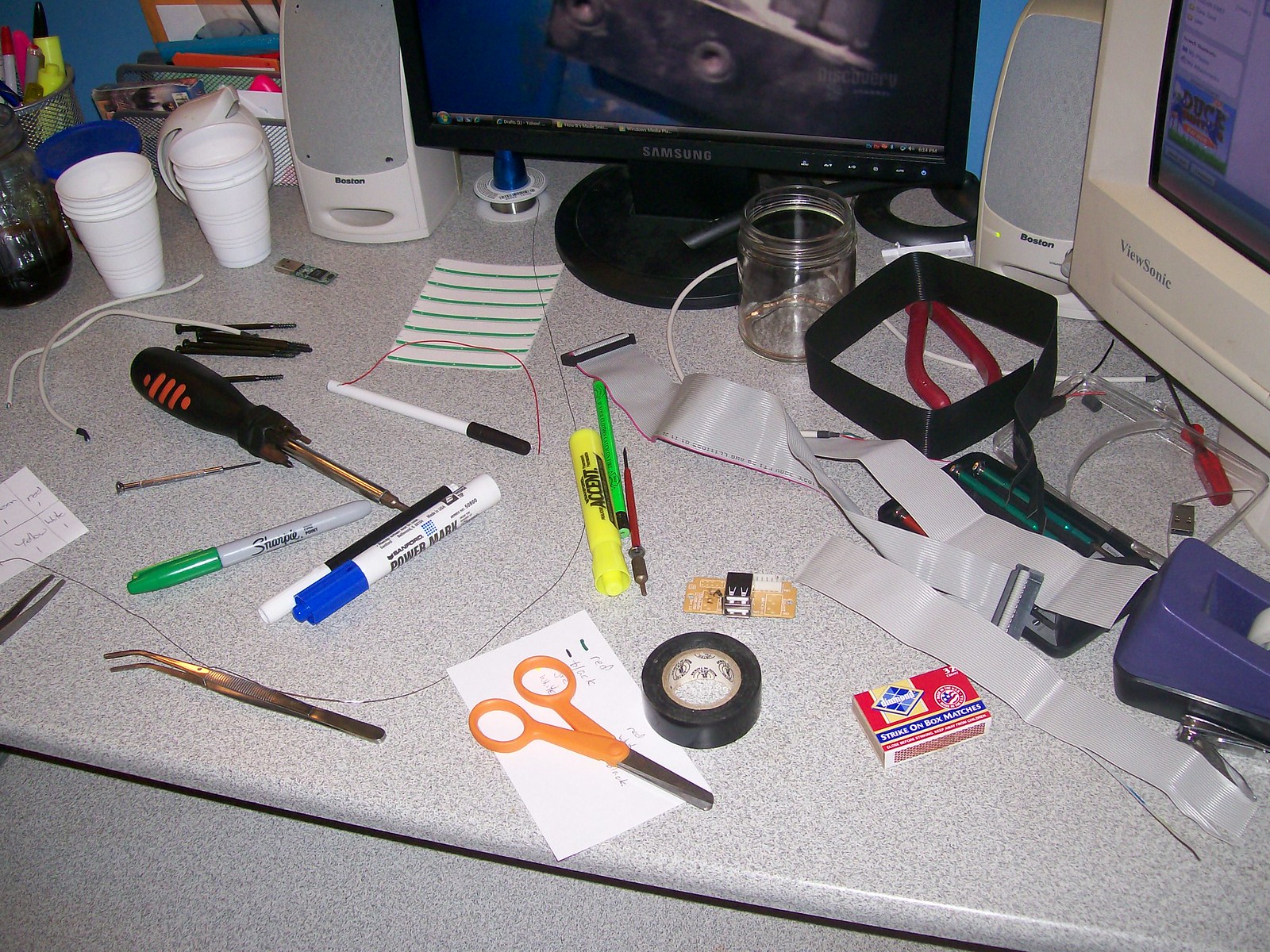This photograph captures the chaotic yet industrious scene of a workspace mid-project. The central focus is a modern Samsung flat-screen monitor positioned towards the middle back of the desk, flanked on the right by an old-style ViewSonic CRT tube monitor. Nestled between these monitors is an antiquated speaker, with another speaker situated to the left of the flat-screen. Moving further left, there's an array of organizational containers holding papers and highlighters. 

In front of these containers, stacks of disposable cups add to the clutter. The gray desk surface is scattered with a diverse assortment of items indicative of an active project. A tape dispenser is positioned to the right, while scissors lie towards the front middle. Nearby, black electrical tape and what appears to be an old chipset or transistor hint at an electronic venture. To the right of this, matches and strips of gray material pulled from a computer—possibly ribbon cables or other internal components—are visible. The surface is further strewn with various tools and supplies: numerous screwdrivers, pens, pencils, highlighters, markers, peelable file labels, tweezers, and assorted wiring are dispersed across the desk. An empty jar also finds a place amidst the organized chaos, suggesting a workspace brimming with activity and purpose.